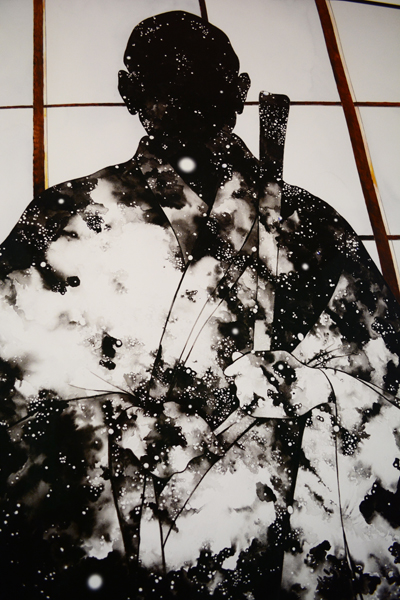This black and white, abstract piece of art features the silhouette of a Japanese warrior in a white belted robe, holding a samurai sword in his left hand. The figure is enveloped in shadow, with only the outlines of his head, hands, and the sword distinctly visible. Dappled light creates patterns of glowing white circles and specks across both the warrior and the gray background. The backdrop consists of a rice paper door with brown wooden frames, divided into rectangular panes. This captivating artwork, with minimal yet precise detailing, brings together elements of traditional Japanese culture and abstract artistic expression.